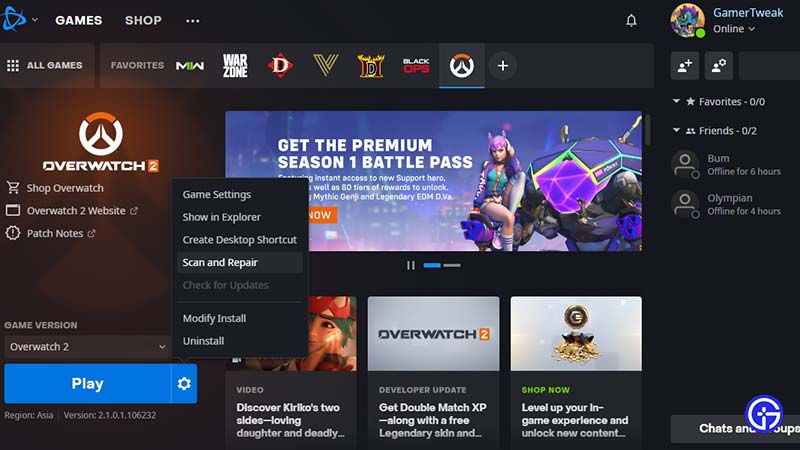The image depicts a gaming shop interface, specifically from a platform named "Gamer Tweak." The profile "Gamer Tweak" is currently online. The dashboard displays various categories, including "All Games" and "Favorites," though it indicates that there are currently zero favorites and two friends online.

A significant portion of the interface is dedicated to "Overwatch 2," featuring several sections such as the shop, website, and patch notices. Prominently, there is a call-to-action to purchase the Premium Season 1 Battle Pass. Additionally, a pop-up window titled "Game Settings" is visible, offering options like "Show in Explorer," "Create Desktop Shortcut," "Scan and Repair," "Check for Updates," "Modify and Install," and "Uninstall." The "Scan and Repair" option is highlighted in white, indicating it's currently selected, while the other options remain greyed out.

In the "Discover" section, there is a feature on "Kiriko’s Two Sides: Loving Daughter and Deadly," along with promotional content for "Overwatch 2," including offers for double match XP and a free legendary item, urging users to shop now and level up their in-game experience to unlock new content.